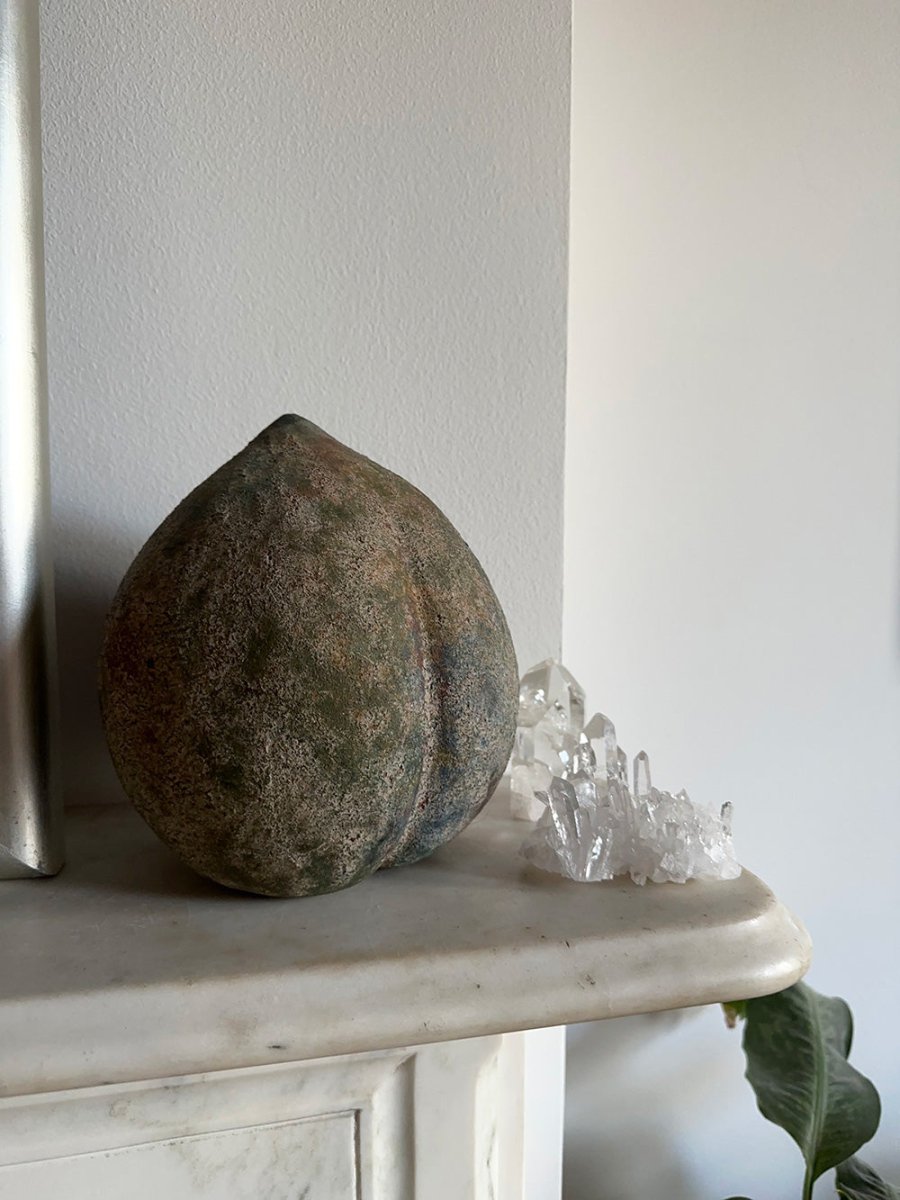A detailed color photograph showcases an elegantly designed indoor setting featuring a marble fireplace mantle adorned with various items. Central to the scene is a large, uniquely shaped black stone, resembling an upside-down peach with a distinctive ridge on its back, marked by orangey, rusty-colored ridges. Beside this intriguing object, to the right, there is a collection of clear white crystals, including a prominent crystal tower and a white geode. The mantle, made of marble with shades of gray, is situated against a gray wall, with a subtle reflection of light casting a gentle glow on a nearby white wall, creating an illusion of separation. Additionally, a single green leaf from a plant is peeking into the frame from below, hinting at the presence of a potted plant just out of view.